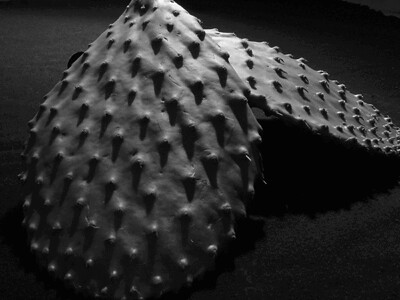This detailed black and white photograph showcases two teardrop-shaped cactus leaves with numerous small, smooth stubs. The composition features one leaf positioned horizontally in the background, pointing to the right, and the second leaf resting on top of it, facing slightly forward and angled partially away from the camera. The leaves appear almost as if the needles were deliberately removed, adding to their rough yet stub-laden texture. Illuminated from above, the light casts distinct shadows, especially under the rightward-leaning leaf, enhancing the depth of the image. The stark black background further emphasizes the white, textured nubs on the cactus leaves, creating a striking and evocative visual contrast.